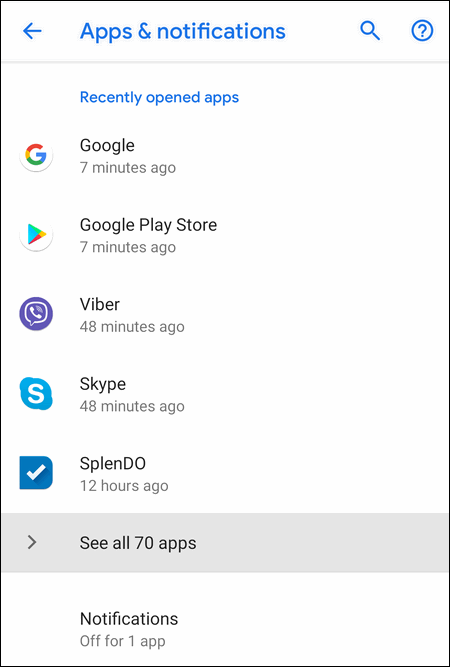The image is a screenshot featuring a table of recently accessed applications. The entire screenshot is encased in a thin black border. At the very top left, there is a left-pointing arrow followed by "Apps and notifications" written in blue. To the right of this text are icons for search and help.

Beneath this, a thin gray line spans the width of the frame. Just below the line, the heading "Recently opened apps" is displayed. There is a list of apps accompanied by their respective icons and the last time they were opened:

1. **Google** (7 minutes ago) - Icon: Google "G" logo.
2. **Google Play Store** (7 minutes ago) - Icon: Play Store triangle.
3. **Viber** (48 minutes ago) - Icon: A phone emitting sound.
4. **Skype** (48 minutes ago) - Icon: Blue diamond with an "S".
5. **Splendio** (12 hours ago).

At the end of the list, there is a gray background bar with a right-pointing arrow and text that reads "See all 70 apps." 

Towards the bottom, there is a white bar stating "Notifications off for one app." 

Each app's logo corresponds to its position, adding visual context to the times they were last accessed.